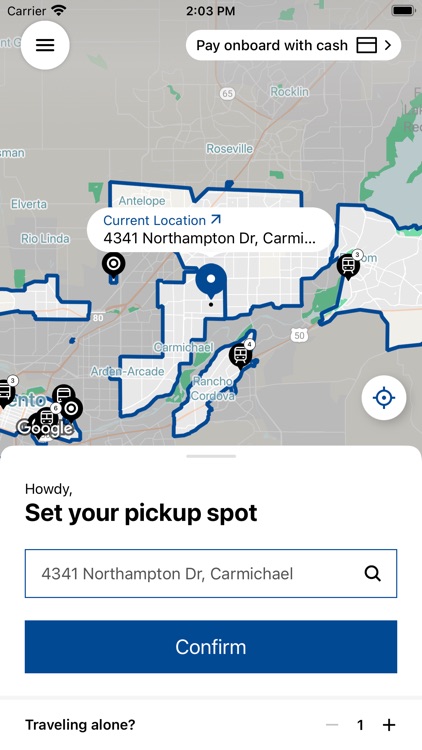The image is a detailed map displayed on a smartphone screen. It features a variety of buttons and information for a transportation service. 

At the top right corner, text reads "Pay on board with cash." Towards the bottom right, a friendly greeting, "Howdy," is shown. Below this greeting, the image prompts the user to "Select your pick-up spot," with the user's pick-up spot already chosen as 4341 Northampton Dr, Kamakia. 

A prominent blue button with white text labeled "Confirm" is located at the bottom center. To the bottom left, text indicates "Traveling alone," and there is a section on the bottom right with controls to increment or decrement the number of people. Currently, it is set to one person.

In the center of the map, several vehicle icons resembling trains are displayed. A blue location pin showing the current location of the requester marks 4341 Northampton Dr, Kamakia. Additionally, a black location pin is visible near the top left of the image. 

The map's background is grey, with white lines indicating roads and blue lines likely representing routes or transit lines.